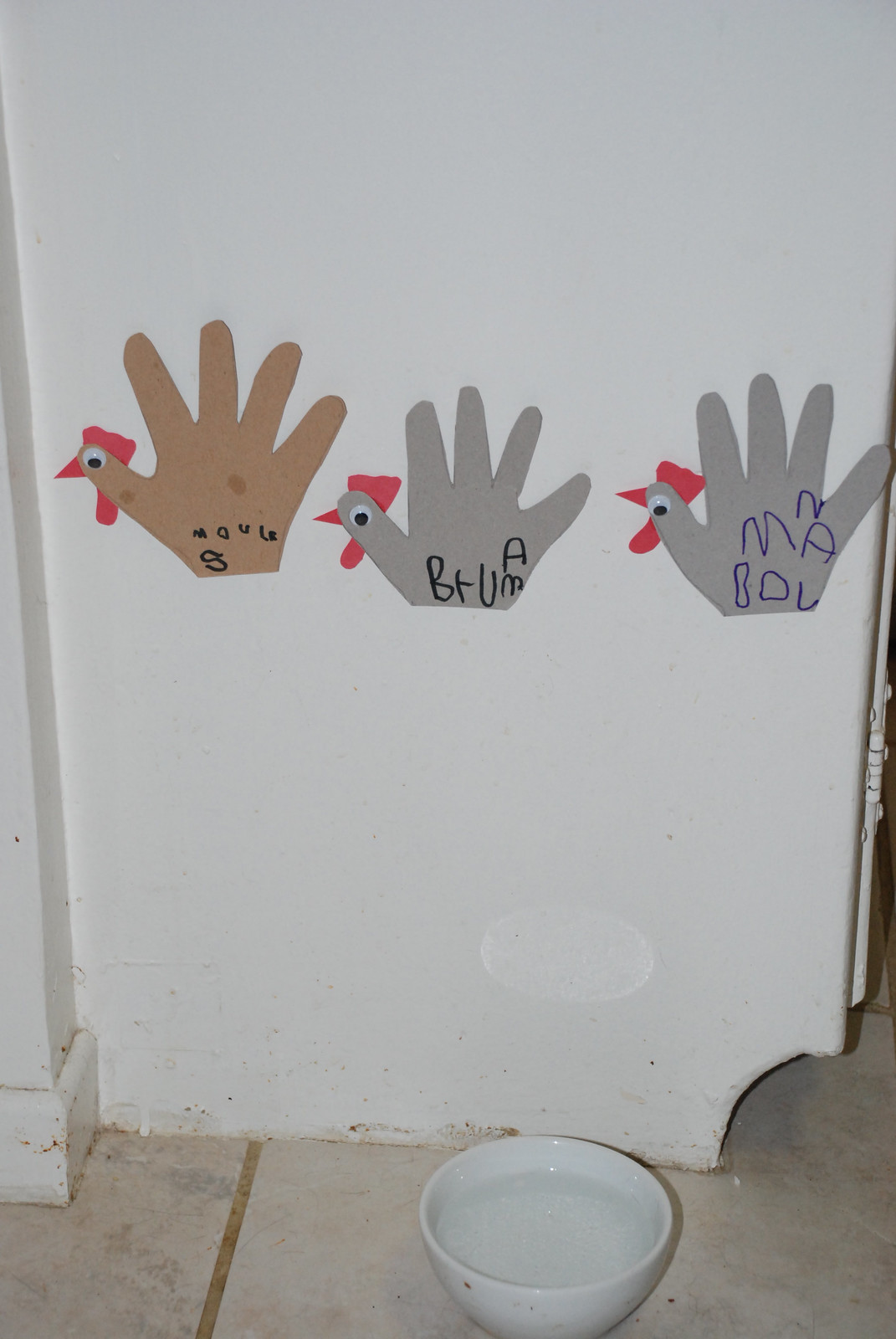The photograph captures what appears to be a slightly damaged section of an old, white wall or possibly a refrigerator, with a noticeable chunk missing from the bottom right corner. The wall stands against a tan, somewhat worn, and dirty tiled floor. Positioned in front of this wall is a white bowl containing water. Centered on the wall are three hand turkey crafts, made by children. Each turkey is crafted from construction paper with their hands traced and cut out, featuring a red head and googly eyes on the thumb to represent the turkey's face. The left hand turkey is brown with the word "MOULS" written on it. The middle hand turkey is grey and has "VRUMA" written in the center. The right hand turkey, also grey, is labeled with the word "MBOLAN." These colorful and whimsical crafts are affixed horizontally, adding a touch of creativity and innocence to the scene.